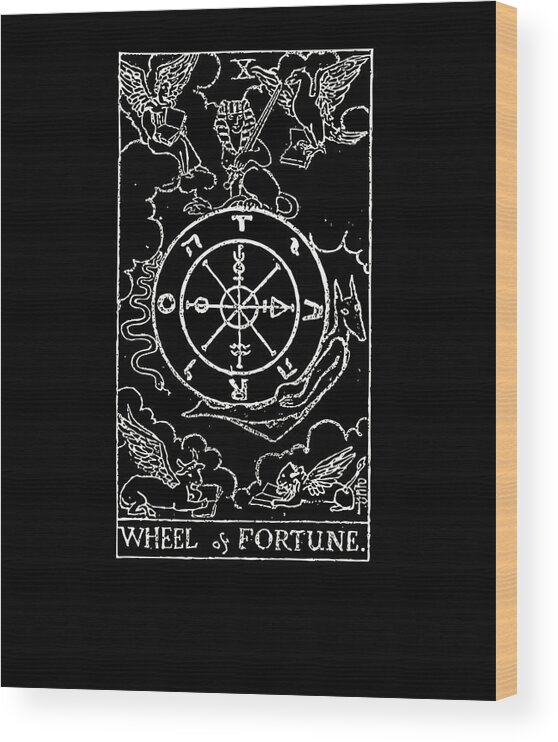The image is a detailed depiction of the cover of a book, prominently featuring a black background with elaborate white line art. At the forefront of the cover is an intricate mural resembling the Wheel of Fortune tarot card, rendered in a black and white palette. Central to the piece is a large circle adorned with cryptic lettering: a 'T' at the top, 'A' at the 3 o'clock position, 'R' at the bottom, and 'O' at the 9 o'clock position, collectively spelling out "TAROT." Surrounding this central wheel are various zodiac symbols and signs, arranged in a circular pattern, with sundials in the center. The top portion of the mural displays mythical creatures, including a Pegasus-like winged horse and two dragons, one on each side. The very top center of the mural bears the Roman numeral 'X', signifying the number 10. At the bottom of this intricate artwork, the words "Wheel of Fortune" are clearly inscribed. The entire composition is reminiscent of a tarot card designed on a wooden canvas, meticulously painted black to highlight the white sketches, creating a stark and mystical visual effect.